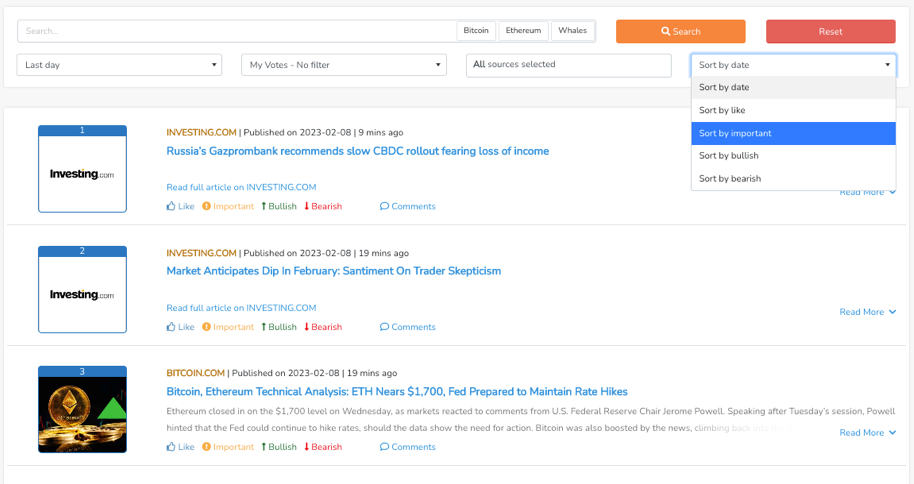The image depicts a complex layout of multiple rectangles and squares, each outlined in light gray or blue. Starting from the left, there are two small squares that are blue at the top and outlined in blue. Both squares contain the text "Investing..." Next to these squares is another square with a blue top and a picture in black and orange, accompanied by a green triangle pointing upward. Below this picture, there are words in gold and black, followed by words in blue, black, and additional colored symbols and text.

On the right side of the image, there is a series of rectangles lined up vertically. The first is a light gray-outlined rectangle. Adjacent to it on the right is another light gray-outlined rectangle containing a word that is unclear. Further to the right, there are three words separated by lines, but their exact text is indistinguishable. Below these elements is an orange rectangle with a magnifying glass icon and the word "Search," followed by a red rectangle with unreadable text.

Moving downward, there is another gray-outlined rectangle labeled "Last Day," followed by another similarly outlined rectangle displaying the text "My Boat, No Filter." Below that, another rectangle reads "All Sources Selected." Adjacent to these, a blue-outlined section appears on the top and sides, indicating "Sort By Date," with the same text repeated below it. Following this, it states "Sort By Light," and there is a blue rectangle that reportedly reads "Sort By Important." Another gray-outlined rectangle is labeled "Sort By..." with unreadable text, followed by an additional gray rectangle labeled "Sort By..."

Finally, encapsulated within these elements are words in different colors, including gold, black, and blue, followed by various symbols. This pattern is repeated, showcasing a detailed and organized yet bustling interface.